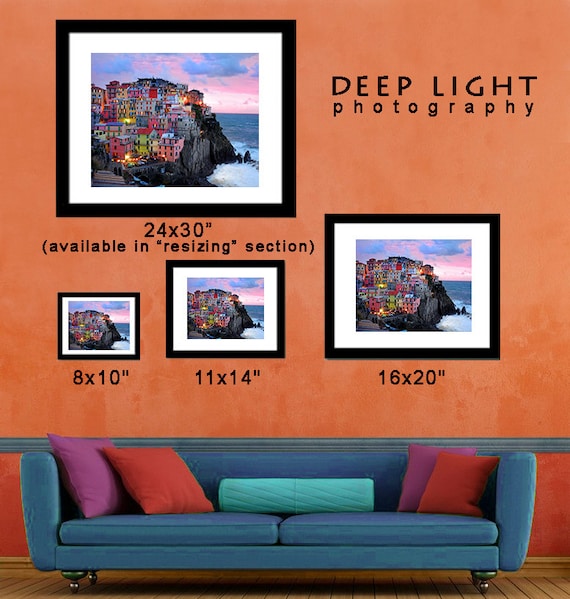The advertisement image showcases a living room with a prominent blue couch at the bottom, featuring two long, thin cushions and five pillows—two purple, two red, and a central blue roll pillow. The wall is painted a bold orange with a brighter orange wainscoting beneath it. Displayed on the wall are four identically framed photographs of picturesque cliffside homes from the Ligurian Riviera, each in a black frame. On the upper left, "Deep Light Photography" is written, followed by "24x30 inches, available in resizing section." Below it are three other framed photos with respective dimensions: 8x10 inches, 11x14 inches, and 16x20 inches. This setting highlights the various available frame sizes for the artwork.